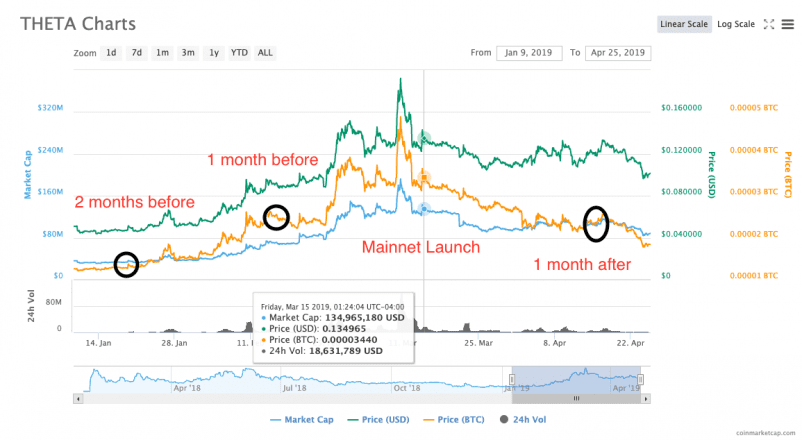**Descriptive Caption:**

The screenshot is of a cryptocurrency analysis tool displaying "Theta Charts" as indicated at the top left corner. In the top right corner, there are options for toggling between a linear and logarithmic scale, accompanied by a maximize button and a menu button for additional settings. Below these, there's a zoom menu offering various time-frame options such as 1 day, 7 days, 1 month, 3 months, 1 year, year-to-date, and all-time, along with fields to input or display specific dates.

The main chart visualizes the market cap and price trends of a specific cryptocurrency from early January to late April 2019. The chart provides comparative data in both U.S. dollars and Bitcoin. Throughout the displayed period, the coin's market capitalization fluctuates within the low 100 million range, while its price oscillates between approximately 4 to 12 cents.